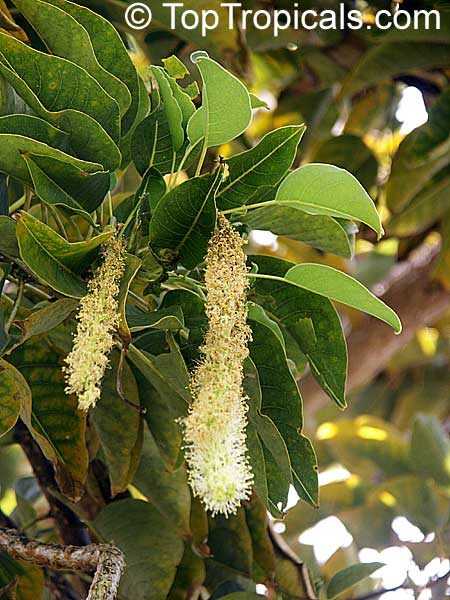The image is a detailed close-up photograph of a piece of vibrant green vegetation, featuring a cluster of leaves and teardrop-shaped flower bundles. The leaves are prominently vibrant green, with some darker ones in the background, and they exhibit a classic leaf shape: curved on the sides and pointed at the ends, supported by a light green central spine.

Central to the image are two hanging bundles of flowers resembling tempura shrimp in texture and form. These bundles are light green to grayish-tan, with some white where the light hits them, giving them a fuzzy appearance due to multiple little stems sprouting out. The larger bundle hangs prominently in the middle of the photo, while a smaller, less healthy-looking bundle is situated to its left, both descending from the stems.

In the background, additional leaves and a hint of sky and light can be seen, although they are out of focus. At the top of the image, the text "toptropicals.com" is clearly visible, indicating the source of the photograph.